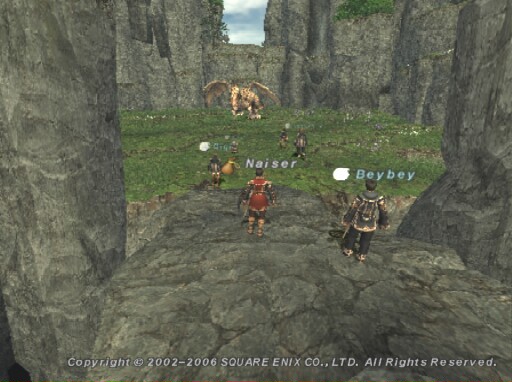In this screenshot from a gameplay, clearly marked with "© 2002-2006 SQUARE ENIX CO., LTD. All Rights Reserved" at the bottom, you see a vivid scene dominated by a rocky landscape surrounding a central grassland. Nestled behind the lush grass, a dragon-like creature sits menacingly. Amidst this setting, there are approximately five characters, three to four of whom are positioned on the grassy terrain while two others stand on the rocky outcrop. Text labels "NAISE" and "BAYBAY" appear above two of the figures on the rocks, indicating their names. The detailed environmental textures and character placements create a rich and immersive gaming world.